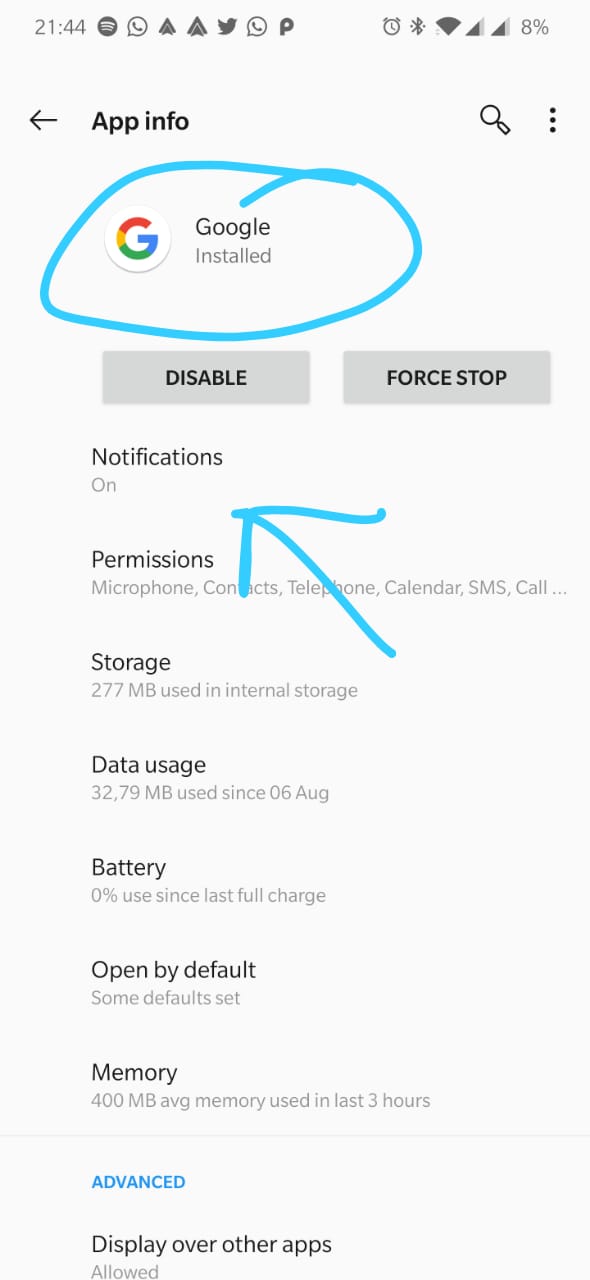This screenshot appears to be from an Android smartphone, as indicated by the numerous timestamps and signal indicators at the top. The background color is a very light gray, almost white. At the very top of the screen, the timestamp is displayed in dark gray text, showing "21:44." Numerous icons are visible, including one with three white lines, a text message symbol, a phone icon, two icons resembling a tent, a Twitter icon, another phone icon, and a "peep" icon. Additionally, the top right corner displays an alarm clock, Bluetooth symbol, full Wi-Fi signal bars, and two signal bars, along with an 8% battery indicator.

The screenshot shows the "App Info" page for the Google app. At the top left, it reads "App info" with a left-facing arrow. On the top right, there are search and more options buttons. Below, the Google app is represented with its white icon featuring the multi-colored 'G'. The text "Google" and "Installed" are displayed beneath the icon. Two gray buttons labeled "Disable" and "Force stop" are also visible.

A hand-drawn teal circle emphasizes the Google icon, with a teal arrow pointing toward the notifications section located below the "Disable" and "Force stop" buttons. The section lists various permissions including microphone, contacts, telephone, calendar, SMS, and storage. It states that the app uses 277 MB of storage and has used 32.79 MB of data since August 6. Additional details include battery usage, default settings, and memory usage. A blue "Advanced" button is located at the bottom of the screen.